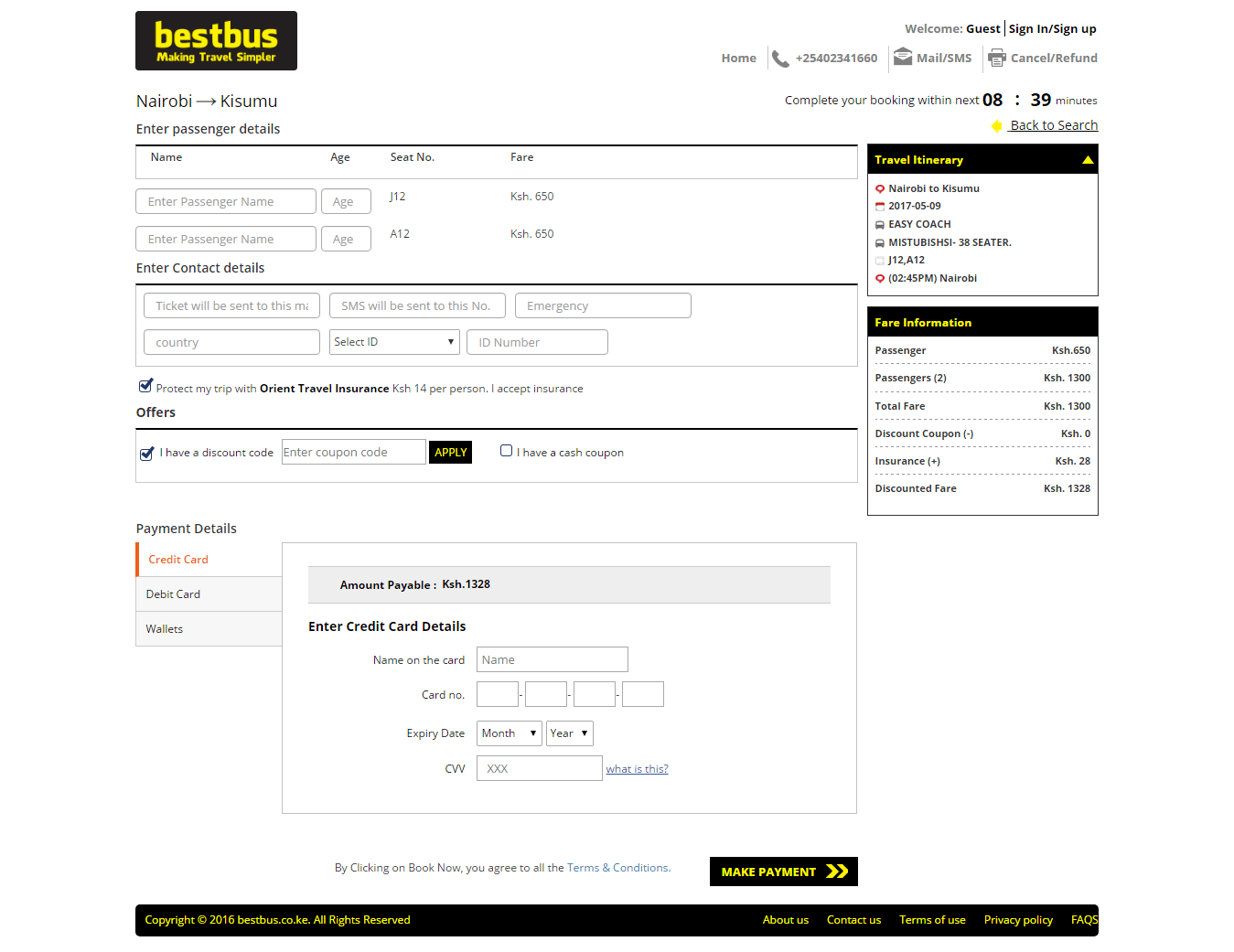The image is an intricate bus ticket or booking confirmation layout with multiple detailed sections. Here's a structured and detailed caption:

---

The upper left corner of the image features a black rectangle with the phrase "Best Bus" in yellow text. Below it, there's an inscription that appears to be "Make Travels," although the text is too small to confirm. On the opposite side of the rectangle are additional words that are illegible due to small font size. Adjacent to these words, there is a sequence of icons. 

The first icon is a phone with numbers next to it, followed by an envelope symbol with accompanying text, and then a printer icon with more text beside it. Directly beneath these elements, the numbers "08:39" are prominently displayed next to a yellow spot with more text beside it. 

Further down the image, there is a section labeled with "Name," "Age," "Seat No," and "Fare," each having corresponding grey-outlined rectangles - two long ones and two shorter ones stacked vertically. Beneath this area, there are several more lines of text followed by a black line, and another set of grey rectangles, totaling six, filled with text that's too small to decipher.

A blue checkmark within a square is positioned underneath, with additional unreadable text beside it. Below this, there's another black line and yet another blue checkmark within a square accompanied by more tiny text. Subsequent to these elements, there's another grey rectangle containing text, followed by a black rectangle with yellow writing.

The layout continues with another grey-outlined square with text beside it. This text segment is followed by more black text with an orange line above it and orange text below. Next, there are two grey rectangles separated by a line, containing more text. Additionally, there’s a white rectangle outlined in grey, topped with a grey rectangle filled with text and further text beneath it.

The bottom segment of the image features further text in black, alongside another grey-outlined rectangle intended for information input. Lastly, at the very bottom, a black rectangle with yellow text reads "Make Payment," flanked by two arrows pointing to the right. This is followed by another long black rectangle at the base of the image, filled with small, unreadable yellow text.